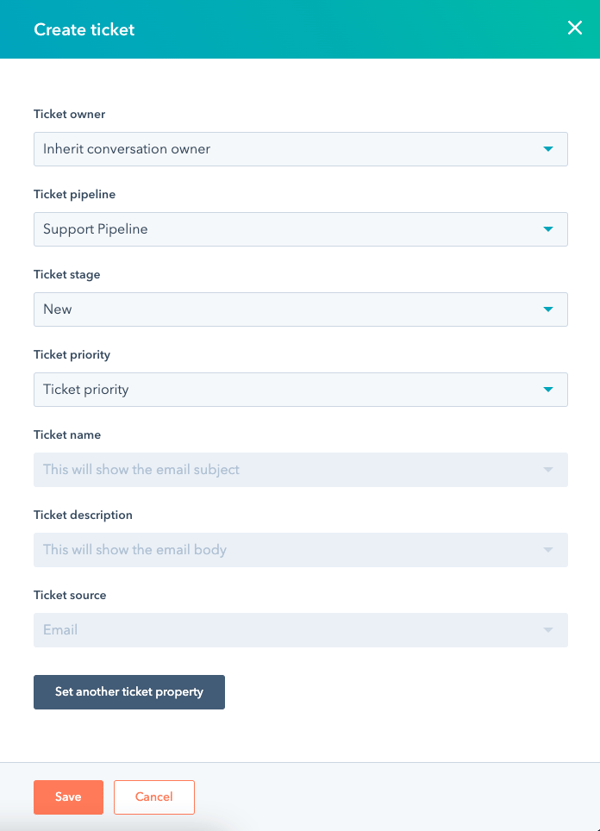A screenshot of a ticket creation form is depicted, featuring various fields set against a blue-green background header stating "Create Ticket." The form is organized with the following elements in black font:

1. "Ticket Owner" with a dropdown box displaying "Inherit Conversation Owner."
2. "Ticket Pipeline" accompanied by a dropdown box showing "Support Pipeline."
3. "Ticket Stage" with a dropdown box reading "New."
4. "Ticket Priority" alongside a dropdown box labeled "Ticket Priority."
5. "Ticket Name" with a notice in the dropdown box indicating "This will show the email subject."
6. "Ticket Description" with an explanatory dropdown box stating "This will show the email body."
7. "Ticket Resource" with a dropdown box that specifies "Email."

Below these fields, there is a dark blue button labeled "Set Another Ticket Property," followed by an orange button that says "Save," and a white button with orange text that reads "Cancel."